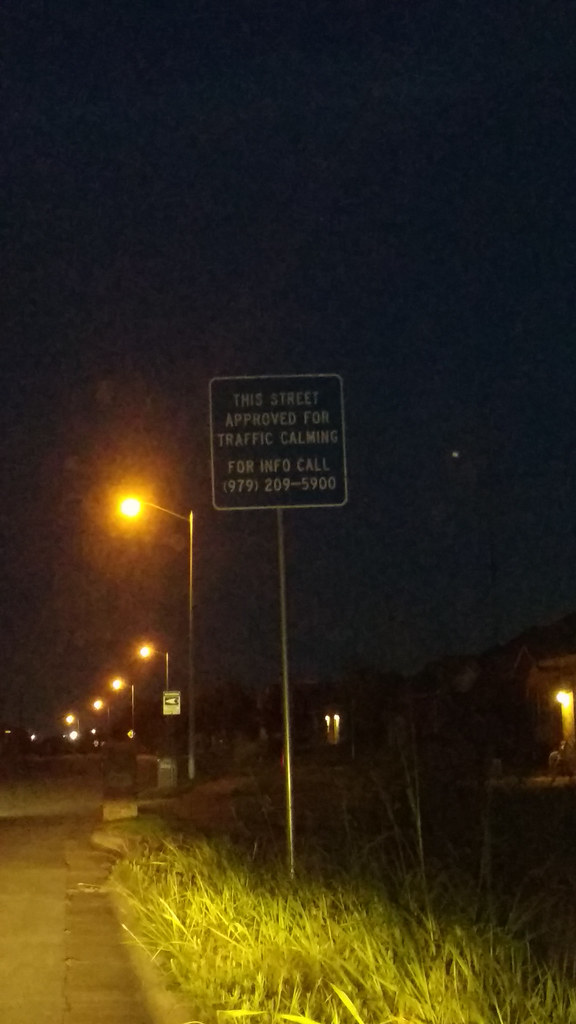In this nighttime photograph, a dimly lit street stretches into the distance, marked by evenly spaced streetlights casting a warm glow against the pitch-black sky. On the left side of the street, tall green grass lines the sidewalk, adding a touch of nature to the urban setting. A prominent black sign with white writing stands amidst the grass, reading: "This street approved for traffic calming. For info call 979-209-5900." Further down the road, another sign is faintly visible on one of the streetlight poles, likely a crime watch sign featuring an eye symbol. In the background, several houses can be seen, their presence indicated by illuminated front porches and glowing windows, though details of their structures remain obscured by the darkness.